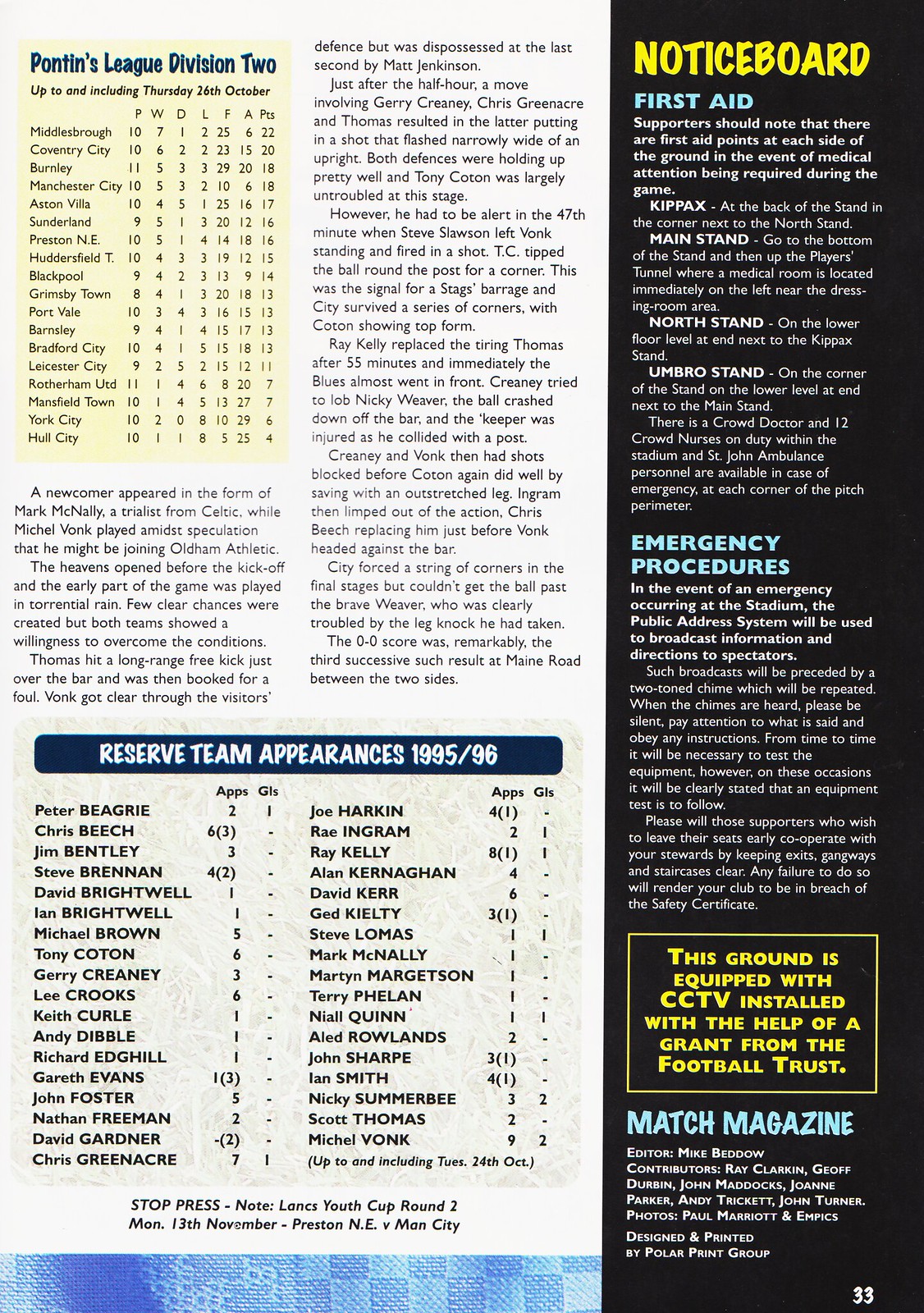This image is a scan of a page from Match magazine, particularly page 33. The page is dedicated to information about the Pontins League Division 2 and includes various sections, each with distinct background colors: beige, pale blue, and black. 

At the top left, within a rectangle that's slightly taller than it is wide, there is a beige section titled "Pontins League Division 2," followed by several paragraphs of related information. The middle section, against a white background, continues with additional paragraphs of text, and includes tables at both the upper left and lower left corners. The table at the bottom left, titled "Reserve Team Appearances 1995-96," contains a list of approximately 40 names along with columns indicating their appearance data.

On the right third of the page, a vertical black banner spans from top to bottom, titled "Notice Board" in yellow letters at the top. This section provides details on first aid locations around the stadium, noting areas such as Kippex, Main Stand, North Stand, and Umbro Stand, and mentions the existence of first aid points for medical attention. Additionally, it includes emergency procedures, stating that information and directions will be broadcast via the public address system in case of an emergency. At the bottom of this banner, there's a yellow box that announces the presence of CCTV surveillance, funded by a grant from the Football Trust. 

This detailed layout is enriched by the diverse use of color and sections that efficiently segment the varied information provided on this page.